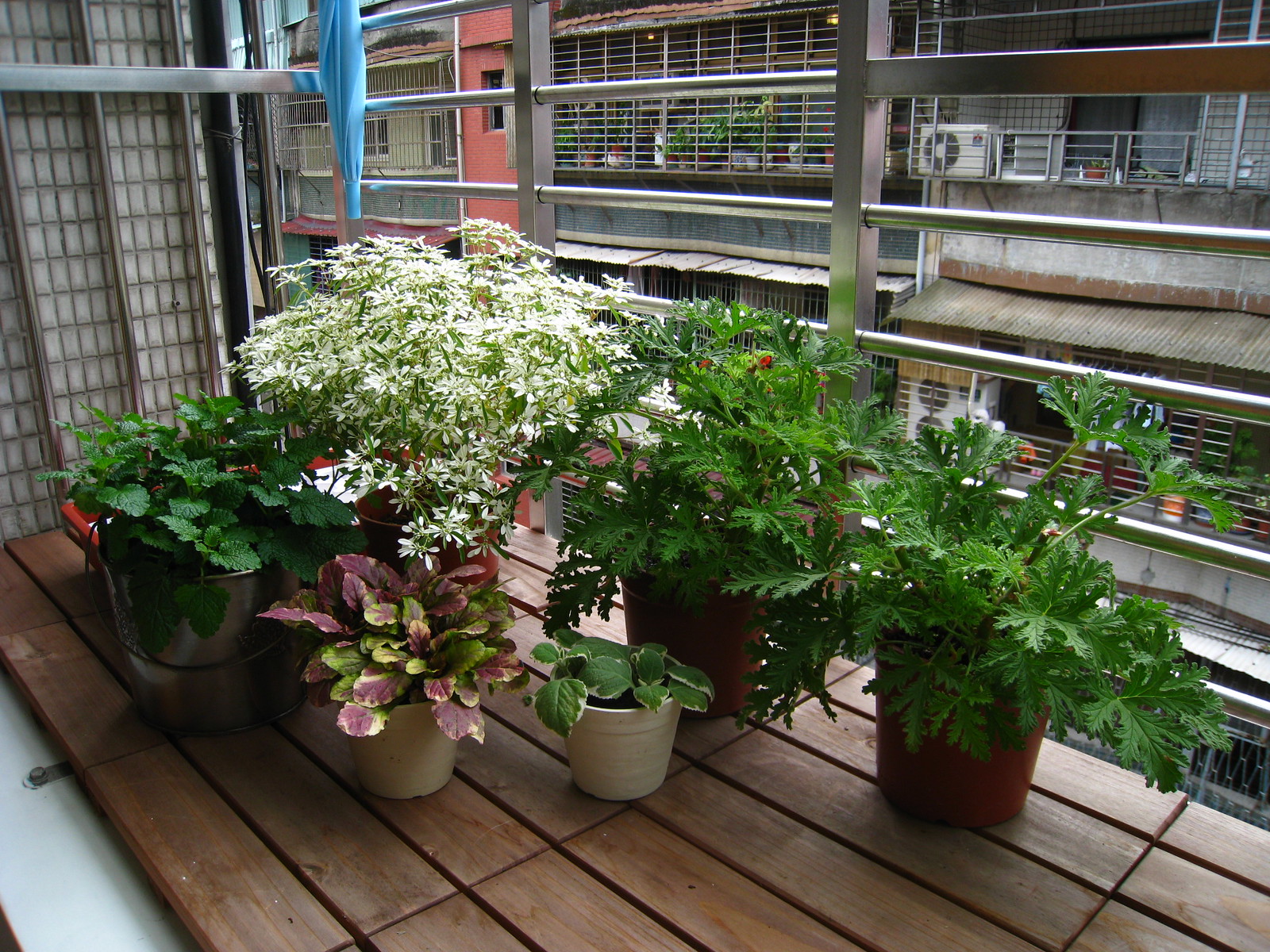This image captures a balcony of an apartment building, seemingly located in a densely built urban area. The balcony features a wooden plank deck positioned on a concrete base painted white. Safety is a priority, evidenced by the metal railing encircling the balcony, a common feature among the neighboring structures. The scene reveals a lively array of potted plants: prominently, two identical red pots housing white-flowering plants, positioned at the front right. Just beside them, two smaller pots display greenery, one with purple leaves and the other with solely green leaves. Additional metal flower pots hold lush green plants, enhancing the verdant appearance. Beyond this balcony, adjacent buildings exhibit barred balconies and varying air conditioning units, suggesting an effort to maintain security and comfort. This bustling alleyway, lined with vibrant greenery and practical utilities, offers a glimpse into the communal and somewhat secure living arrangements, possibly located in an Asian city.